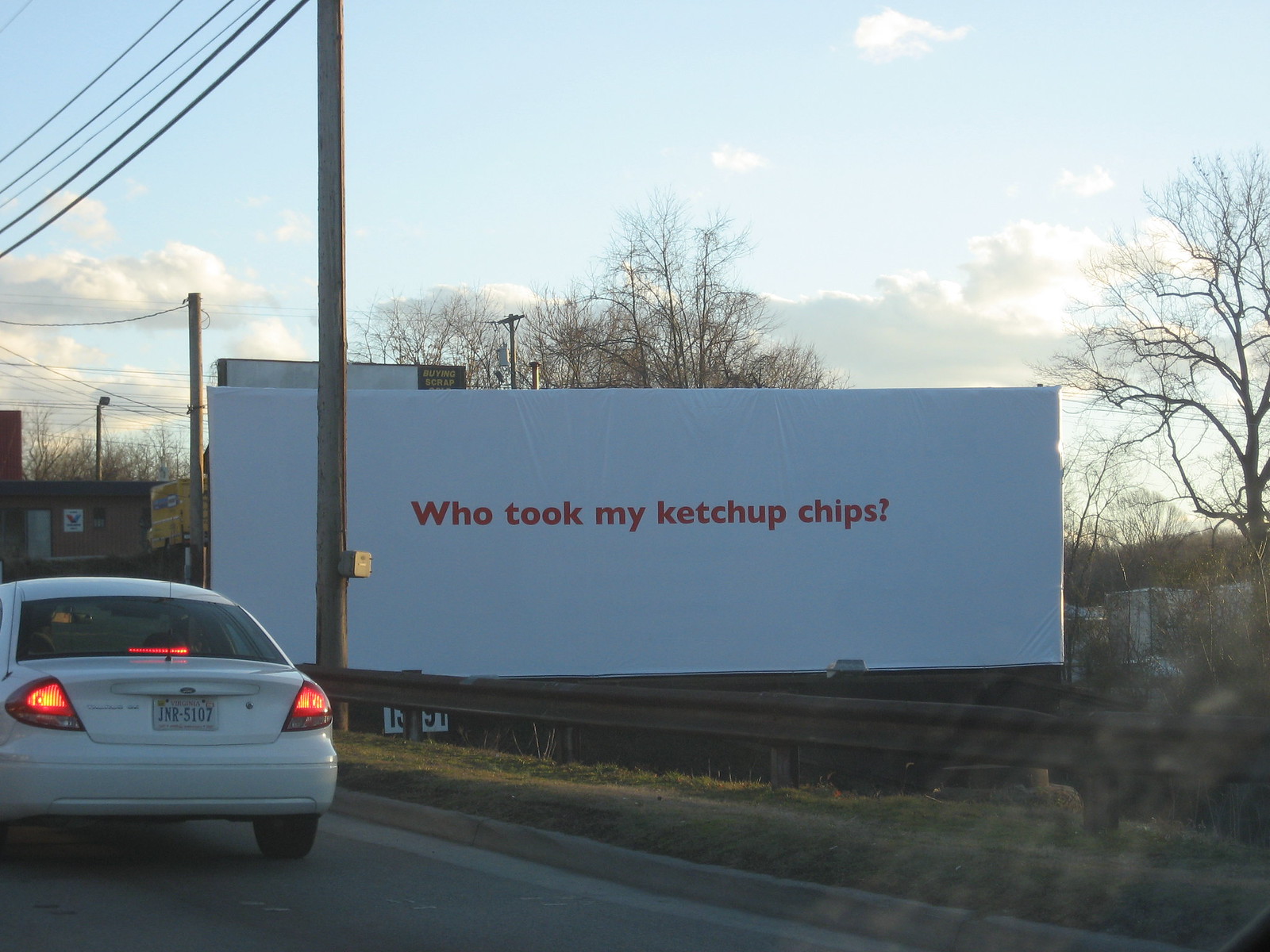A photograph captures a roadside scene under a blue sky with billowy white clouds. In the bottom left corner, there’s a white sedan with its rear backup lights glowing red, positioned on a typical dark brown or black roadway. Diagonally to the right of the car, there’s a sidewalk running parallel to a guardrail. Behind the guardrail stands a large, rectangular white billboard, conspicuously low to the ground. The billboard bears the curious red-lettered message: “Who took my ketchup chips?” On the left side of the billboard, a light post supports several power lines overhead. Above the car, the aged bricks of what appears to be an old factory building stand prominently. The landscape around the billboard suggests it’s winter, marked by a barren stretch of trees and brush devoid of leaves, indicating a stark, almost desolate environment.